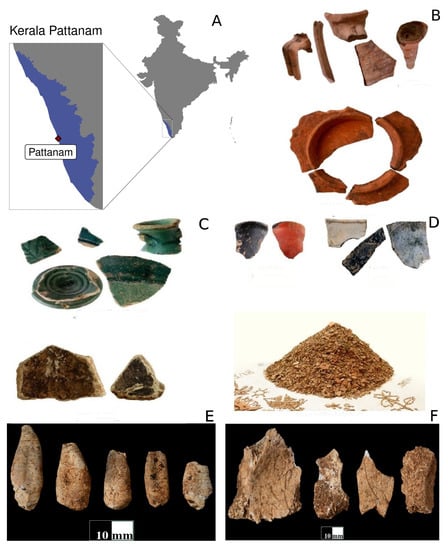The image showcases an organized display of archaeological findings, primarily consisting of pottery shards and fossils, all labeled with letters for clarity. In the upper right, fragments of a brown clay pot are visible, accompanied by grey and green pieces of pottery to the left. Below these, two sections display additional artifacts: to the left, what appears to be stones, and to the right, a mysterious powder. Further below, there are images of ancient stones. A prominent feature in the upper left corner is a zoomed-in map highlighting 'Patanam' in blue, presumably the origin of the artifacts, and another section of the map indicates 'Kerala.' Lettered labels identify different pottery: 'B' for brown, 'C' for green, and 'D' for a mix of black, white, blue, and pink pottery. Additionally, 'E' appears to show an image of shark teeth, accompanied by a scale indicating 10 millimeters for size reference. 'F' contains larger teeth or ground-up substances resembling bone shards. The intricate arrangement underscores a detailed and diverse collection of historical artifacts.